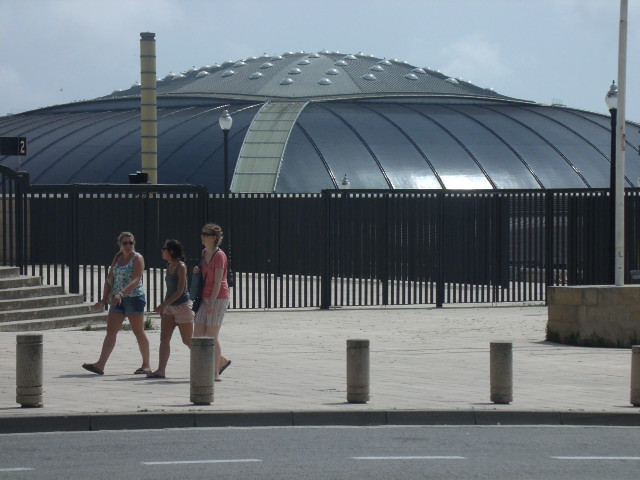The image captures three women walking on the left side of the frame, each wearing dark sunglasses, indicative of warm weather. The trio is moving past the exterior of the Palau Sant Jordi in Barcelona, an iconic indoor arena designed by Japanese architect Arata Isozaki, notable for its dark, curved roof with distinctive center accents. The woman on the right is dressed in a sleeveless green and white tank top, blue jean shorts, and slippers, and she carries a bag. Beside her, the middle woman dons a blue tank top and pink bum shorts, also paired with slippers. The woman on the far left sports a pink t-shirt and shorts with stripes. The setting includes a visible road, lane markings, concrete posts, lamp posts, fences, and the distinctive architecture of the arena, built as part of the Olympic Park for the 1992 Summer Olympics.